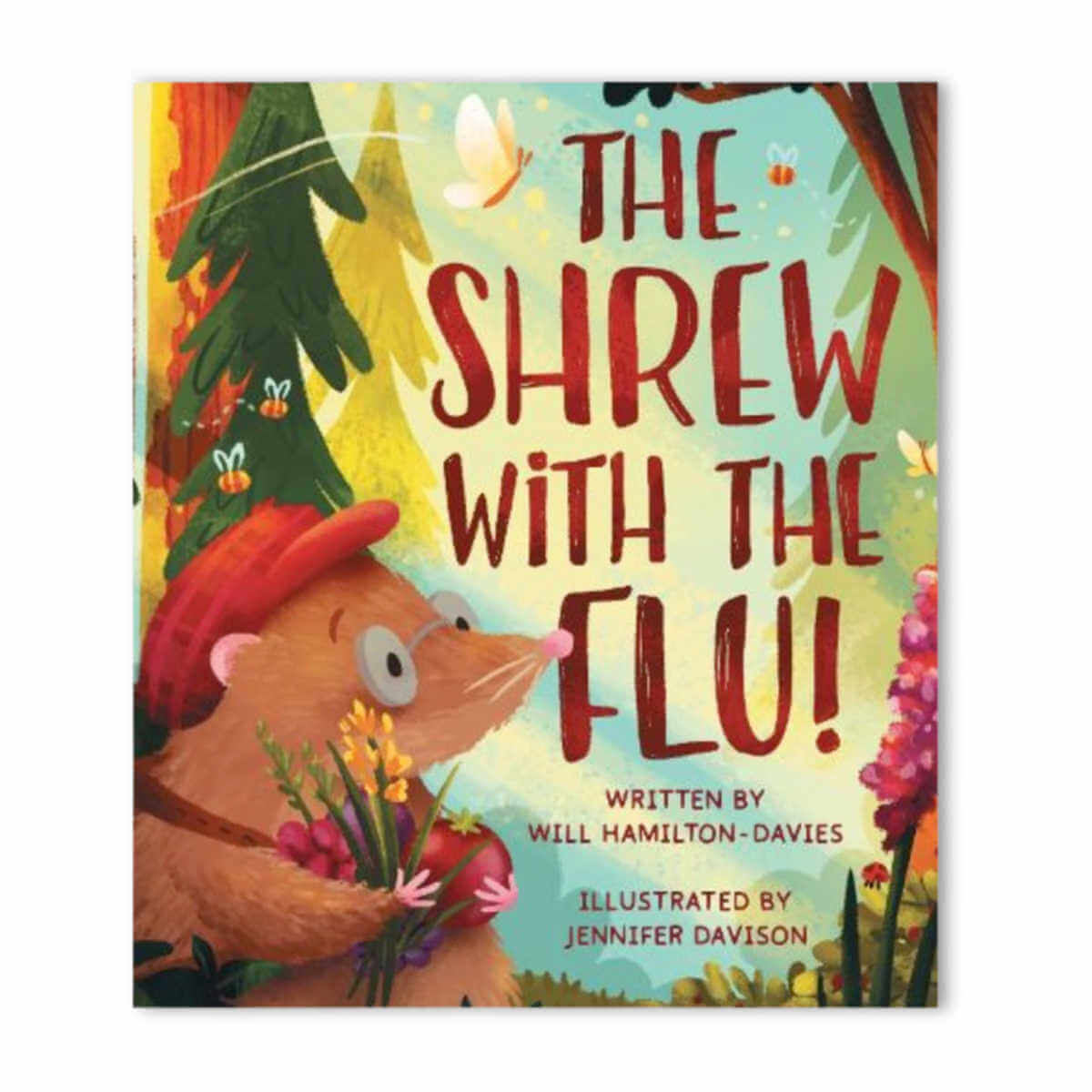The cover of the children's book "The Shrew with the Flu!" features an eye-catching design with bold red text for the title. Below the title, it states in smaller red letters, "Written by Will Hamilton-Davies" and "Illustrated by Jennifer Davison." The cover showcases a whimsical forest scene with tall pine trees and a light sky as the backdrop. In the foreground, a charming brown shrew with beady eyes and circular glasses is depicted. The shrew has a pink nose, little pink hands, and wears a red plaid newsboy cap. It cradles a bouquet of flowers alongside a bright red berry or tomato. Surrounding the shrew, colorful butterflies and buzzing bees add to the lively atmosphere. There are also hyacinths and other assorted flowers scattered around, including some red flowers at the bottom right corner. A ladybug can also be spotted nearby. The overall illustration exudes a vibrant and enchanting feel, perfect for a children's storybook.